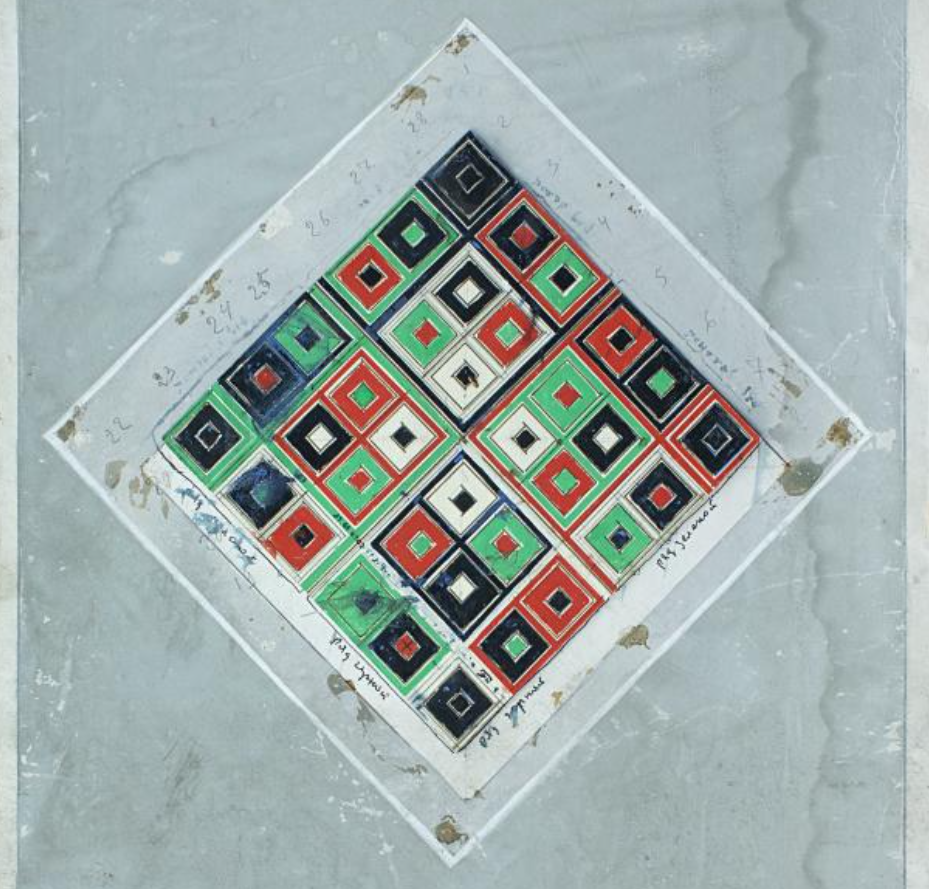The image displays a richly textured, square background with a gray hue, interspersed with darker gray lines and white spots that resemble the appearance of wet paper. In the center, a large diamond shape emerges, bordered by layers of white and various shades of gray. Within this diamond is an intricate mosaic of smaller diamond and square shapes, which are brightly colored in a palette of navy, red, white, and green. The central diamond is divided into four larger sections, each containing six rows and six columns of these smaller shapes. Each smaller square is distinctive; for instance, some have green outlines with blue interiors, others have red outlines with navy and white interiors, and so forth. The layout gives a multidimensional, almost Rubik's Cube-like impression. Additionally, cursive writing, possibly in a foreign language, adorns the outer edges of the square elements, adding an enigmatic touch to the composition.